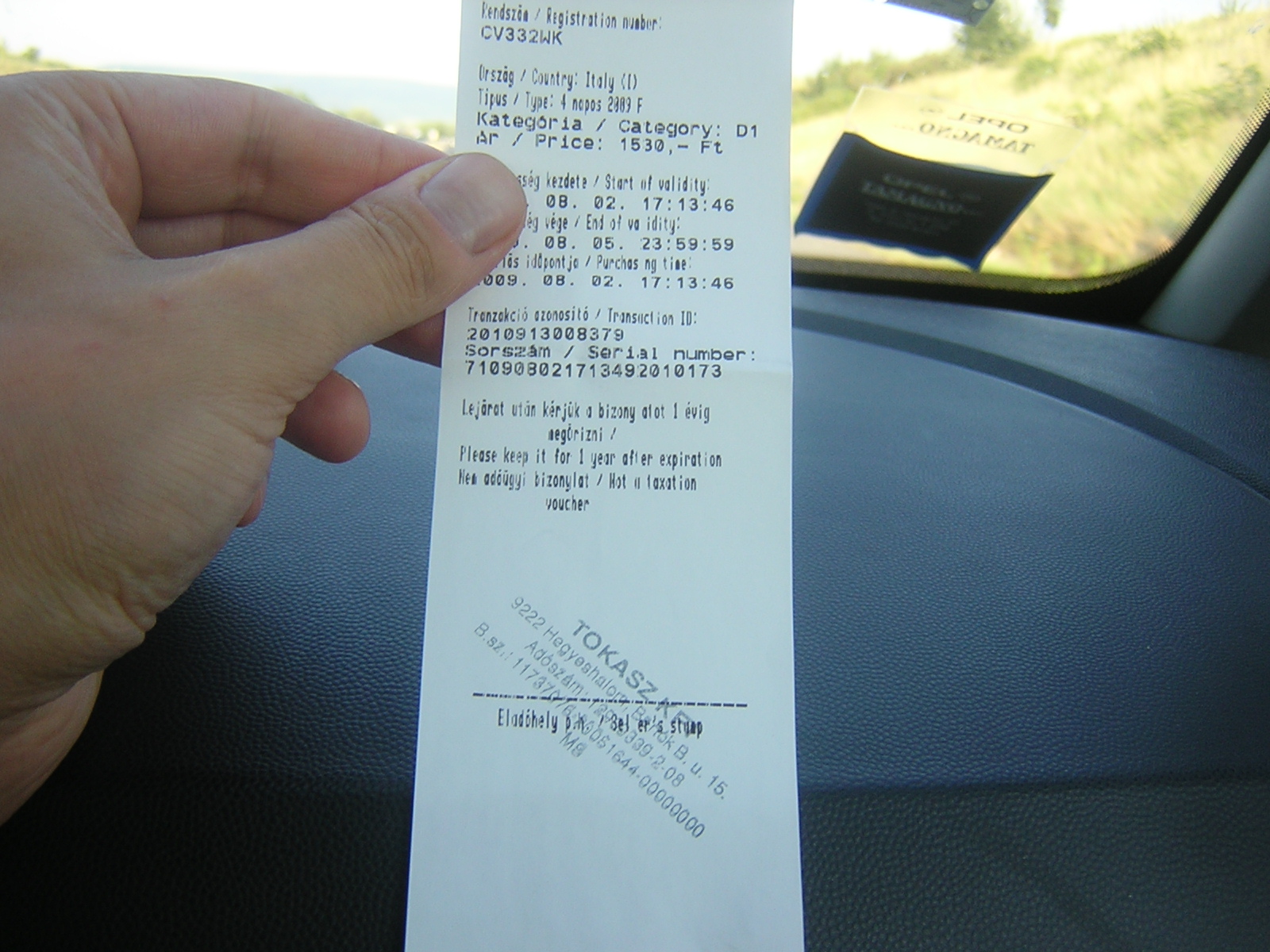In the image, a Caucasian person's left hand is prominently displayed as they hold a white, rectangular receipt between their thumb, index, and middle fingers. The person's fourth finger is partially visible. The scene is set inside a vehicle with a black dashboard. Through the windshield, a gray, overcast sky and a green, grassy incline are visible, suggesting a mountainous area in the background. The windshield also has a rectangular decal located on the lower right-hand corner. The decal is predominantly black with some portion being clear, showcasing black and gold writing that is difficult to decipher. The receipt itself features black text, appears to be in French, and includes various details such as a registration number reading "CV332WK," a reference to "country, Italy," and a price marked as "1530-FT." Near the bottom of the receipt, there is a stamp with partially legible text, including "T-O-K-A-S-Z."